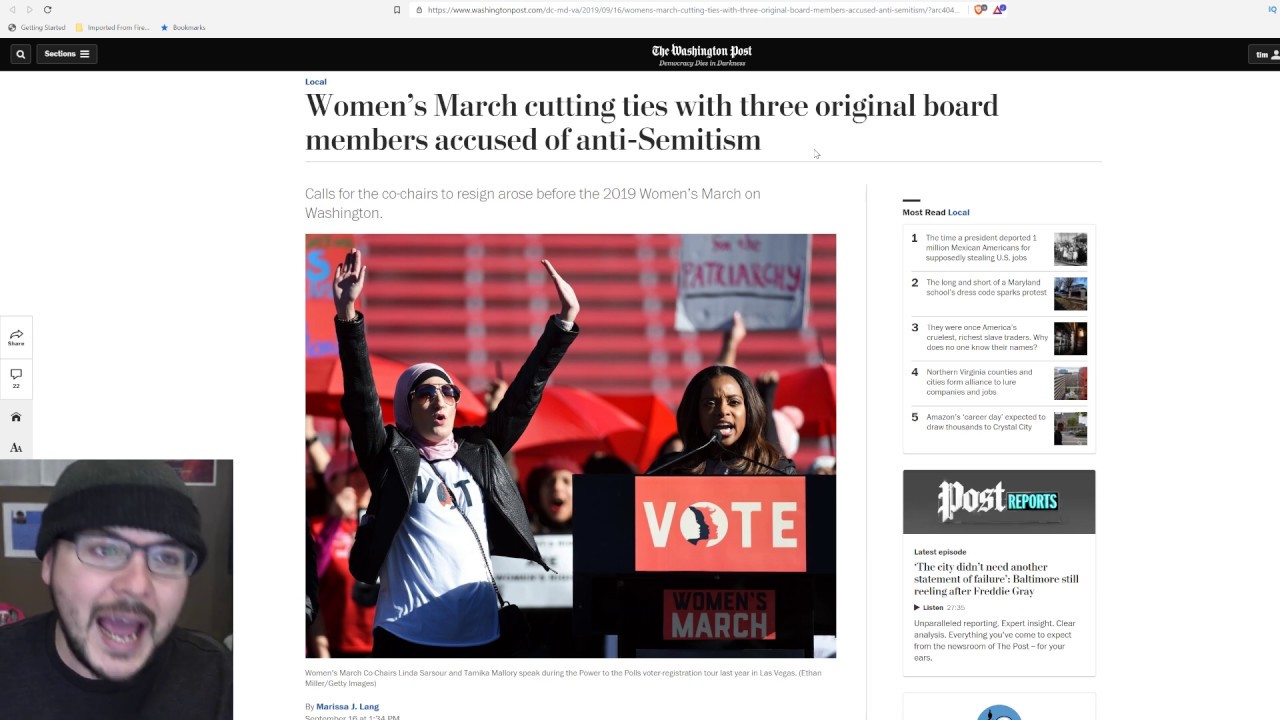The top portion of the webpage features a gray header with the text "Getting Started" followed by the partially visible phrase "imported from Fire." Next to this text is a blue star icon labeled "Bookmarks." Below the header is a white rectangular web browser address bar displaying the URL: "https://www.washingtonpost.com/dc-maryland-va/2019/09/16/womens-march-cut-ties-with-three-original-board-members-accused-anti-semitism/?arc404."

The central section of the page has a black background with the phrase "Washington Post - Democracy Dies in Darkness" written in white text. Transitioning to a white background, the upper left corner features the word "Local" in blue. Just below, in black text, it states the headline: "Women's March cuts ties with three original board members accused of anti-Semitism." The article notes that these accusations have led to calls for the co-chairs' resignation ahead of the 2019 Women's March on Washington. The byline reads "By Marissa J. Lang," with the author's last name possibly being "Long."